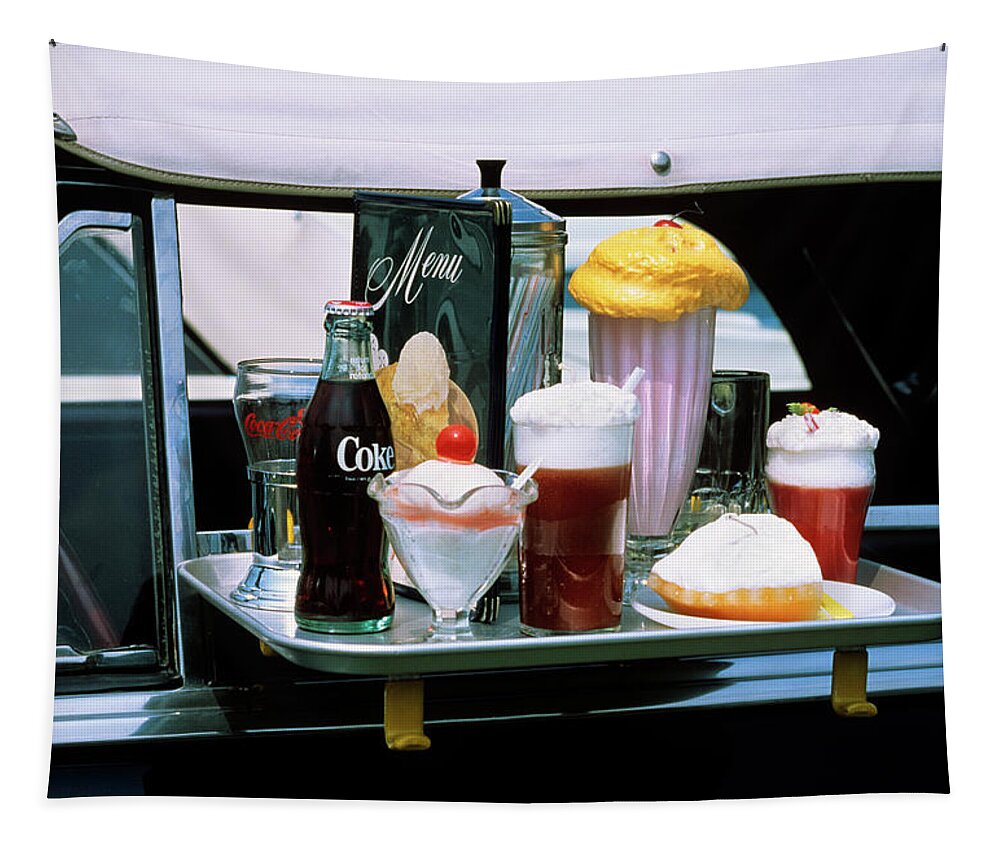This image depicts a vintage 1950s or 1960s dark-colored convertible with a white soft top, featuring a classic doo-wop style drive-in restaurant tray hanging from its window. The silver metal tray is laden with an array of nostalgic treats and beverages. Prominently displayed is an unopened bottle of Coca-Cola alongside a glass bearing the Coca-Cola logo. Also on the tray are a jar with straws, a menu, and a variety of delightful desserts including a sundae topped with a cherry and a root beer float. Several milkshakes, including a strawberry milkshake, complete with straws and whipped cream, add to the assortment. Additionally, there is a plate with a piece of fruit pie, enhancing the scene with inviting red, cream, and pink hues. This charming setup evokes the nostalgic ambiance of the golden era of carhops and drive-in diners.